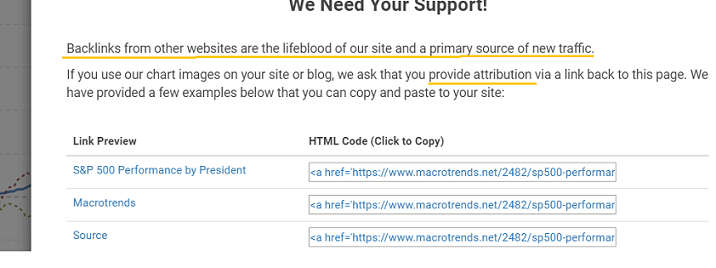This image appears to be a screenshot of a webpage with instructions on how to support the site through backlinks. The background is entirely white with black font. At the top, it prominently displays the phrase "We need your support" underlined in yellow. Below this, the text states, "Backlinks from other websites are the lifeblood of our site and a primary source of new traffic." It further explains that if users incorporate the site's chart images into their own blogs or websites, they are asked to provide proper attribution via a link back to the page. 

To facilitate this, the page provides several code examples for easy copying and pasting. There's a small table consisting of two columns: "Link Preview" on the left and "HTML Code Click to Copy" on the right. The "Link Preview" column features clickable blue text such as "S&P 500 performance by president," "macro trends," and "source," whereas the adjacent column contains the corresponding HTML code snippets that begin with `<a href="https://www.macrotrends.net/2482/sp-500">`.

Additionally, faint dotted lines, resembling maps or chart trends, partially obscured by the pop-up window, can be seen in the background. The left side of the image also shows what appears to be a rolled-up piece of paper with diagrams at the bottom of the third. This detailed arrangement highlights the emphasis on proper citation to enhance the website’s visibility through backlinks.